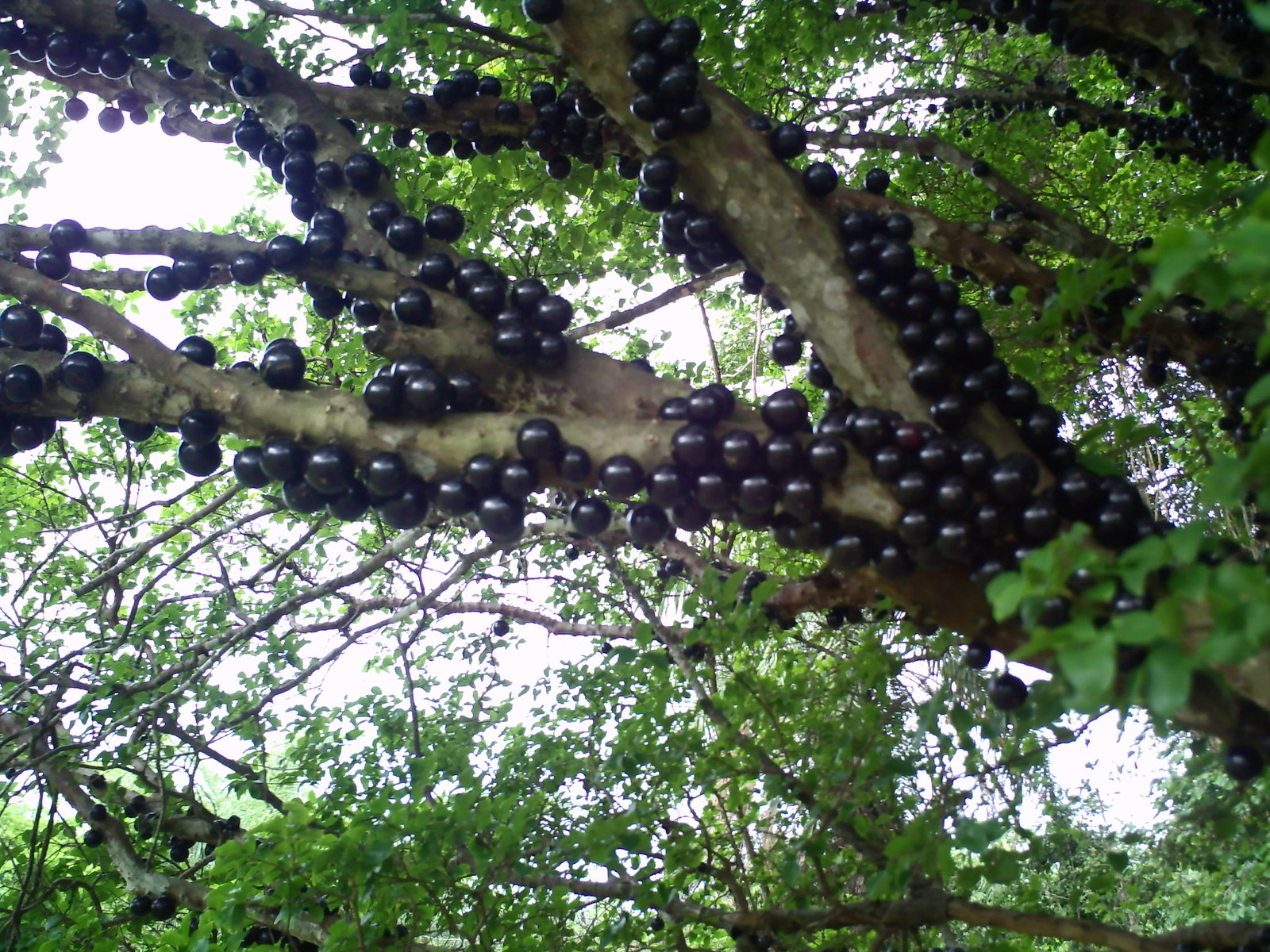The image depicts a tree branch densely covered with numerous black, circular objects growing on its thick wooden parts. These objects, resembling black olives or small apples in size and shape, are perfectly round and appear in abundant clusters throughout the tree. The background reveals more branches with the same black circles, interspersed among a plethora of green leaves. The setting seems to be outdoors in a forest or jungle, hinted by the lush greenery and the clear sky peeking through the gaps in the foliage. The overall color scheme consists of the black circular objects, green leaves, and beige-tan tree limbs. The photograph appears to have been taken during the daytime in a natural environment.